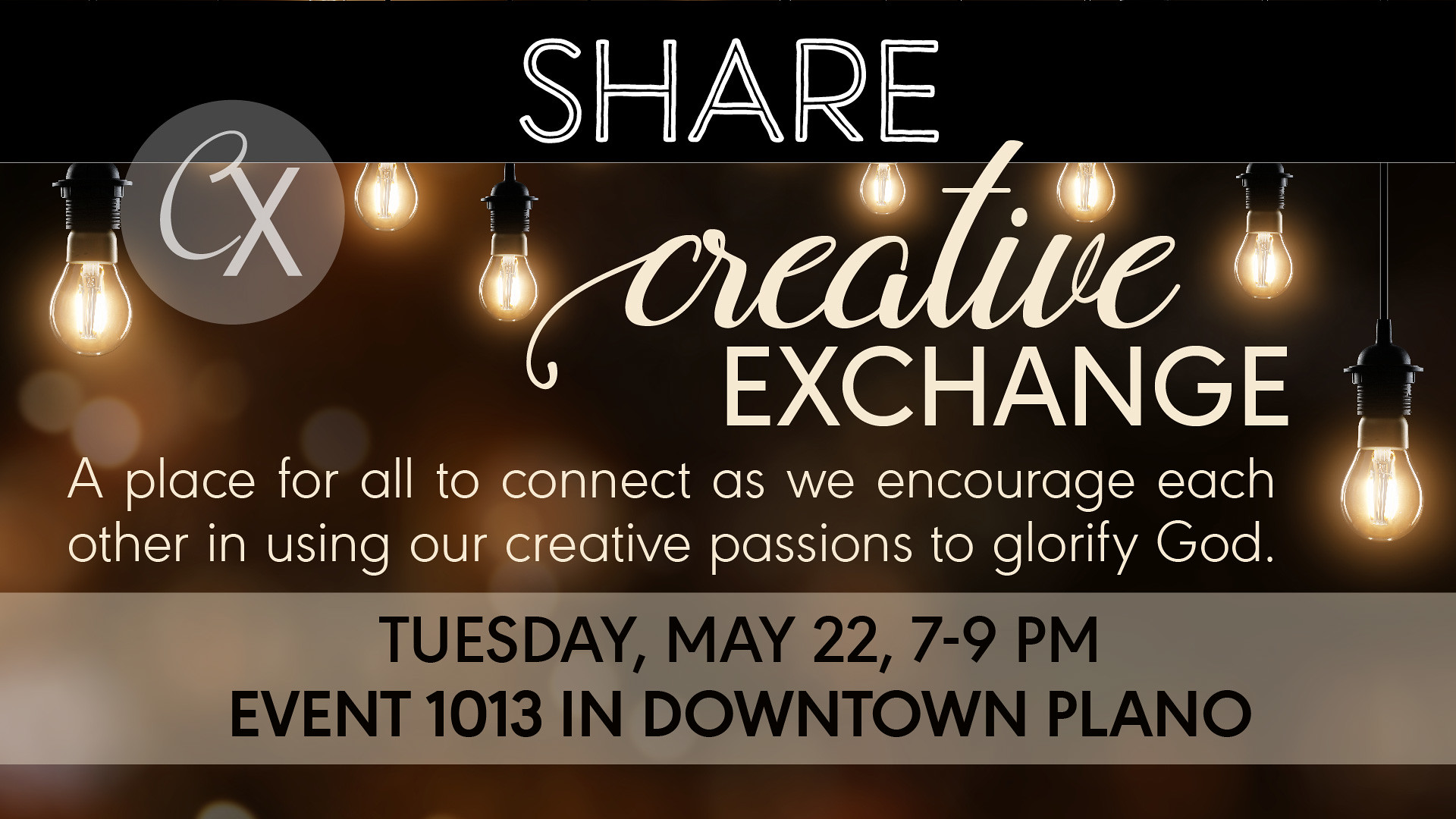The image displays a rectangular landscape advertisement predominantly in shades of black, gray, white, yellow, and tan. The background showcases seven bright, hanging light bulbs against a dark, blurred setting. At the top of the poster, there is a black banner with the word "SHARE" in a white, outline font. To the left of the banner, there's a circular gray logo with the letters "CX" in white script.

Dominating the middle section, "CREATIVE EXCHANGE" is prominently displayed, with "creative" in a lowercase cursive-like font and "EXCHANGE" in bold, uppercase letters. Beneath this title, the text reads: "A place for all to connect as we encourage each other in using our creative passions to glorify God." This message emphasizes the community and religious nature of the event.

At the bottom, a light brownish-gray strip features details about the event in black, all-capital letters: "Tuesday, May 22nd, 7 to 9 p.m., Event 1013 in downtown Plano." The advertisement appears to promote an upcoming religious gathering focused on creativity and connection.